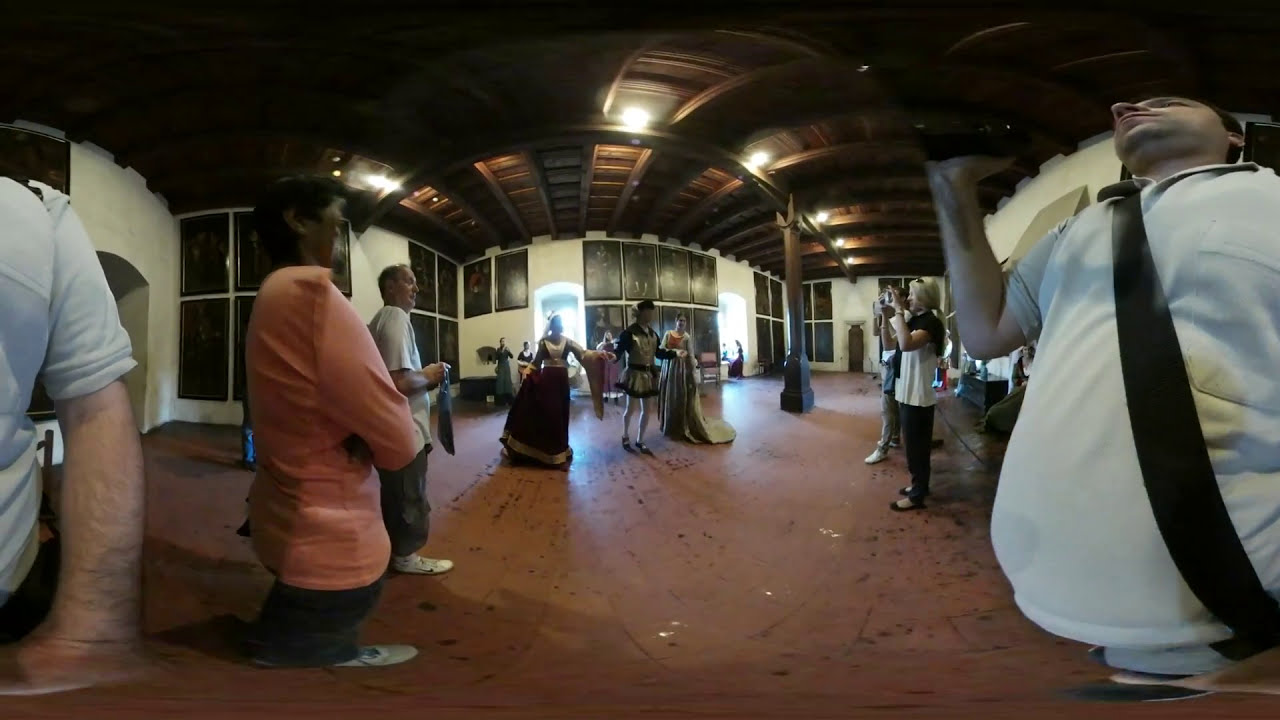The photograph captures a lively scene set in what appears to be a patio or courtyard area, marked by its red or clay-colored floor and ceiling adorned with wooden rafters. The setting is either in front of or inside a building with white walls, decorated with black and white pictures. In the center of the image, three individuals dressed in period costumes reminiscent of old England are the focal point. The two women wear large, elaborate dresses while the man between them is in white tights and a distinctive, possibly kilt-like garment with a peculiar top and an old-style hat. They seem to be performing or possibly dancing while a captivated audience watches. To the right, a line of photographers captures the moment, their cameras raised. Among them, a man with a camera strap over his shoulder is prominently featured in the foreground on the right. Another woman, wearing a salmon-colored shirt, stands with her arms folded on the center left, observing the spectacle.